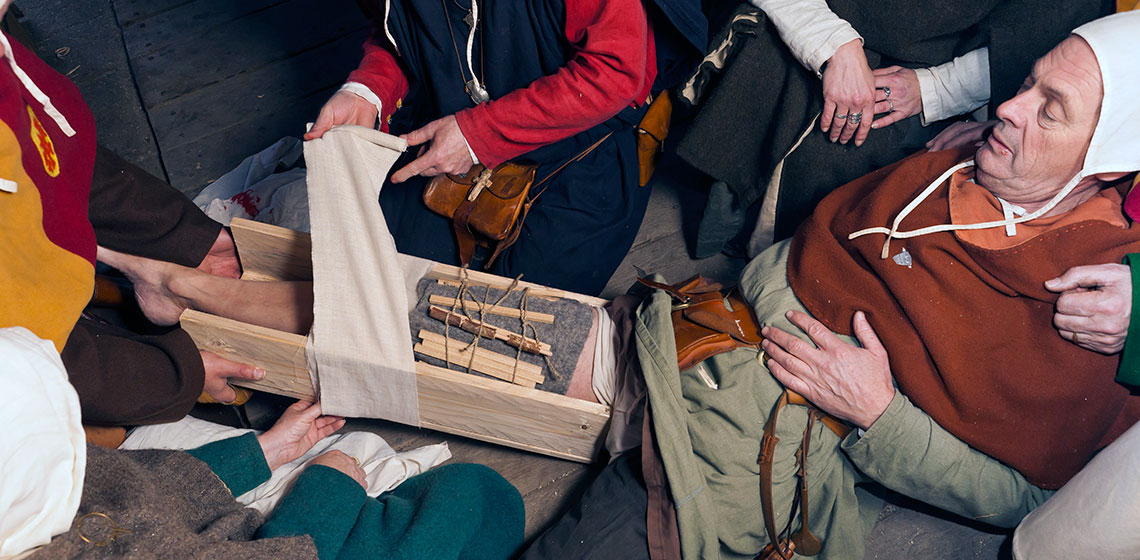The image depicts an older, fair-skinned man with his leg encased in a wooden frame, suggesting he might be an accident victim undergoing a traditional healing procedure. His leg is exposed, wrapped in a grey cloth and stabilized with sticks, while white bandages are being methodically wrapped around the entire setup. The man's attire includes a white headscarf with strings, a brown cowl, and a green robe, indicating a period or Renaissance festival setting. Surrounding him are several figures in period costumes, featuring capes, robes, and leather pouches, although their faces are obscured. One individual kneels beside him, assisting with the bandaging, dressed in a blue robe with red sleeves, and another in a black robe with white sleeves sits close by, displaying rings on their fingers. The scene emphasizes a communal effort in attending to the man's injury, framed by the vivid costumes and accessories emblematic of the era.